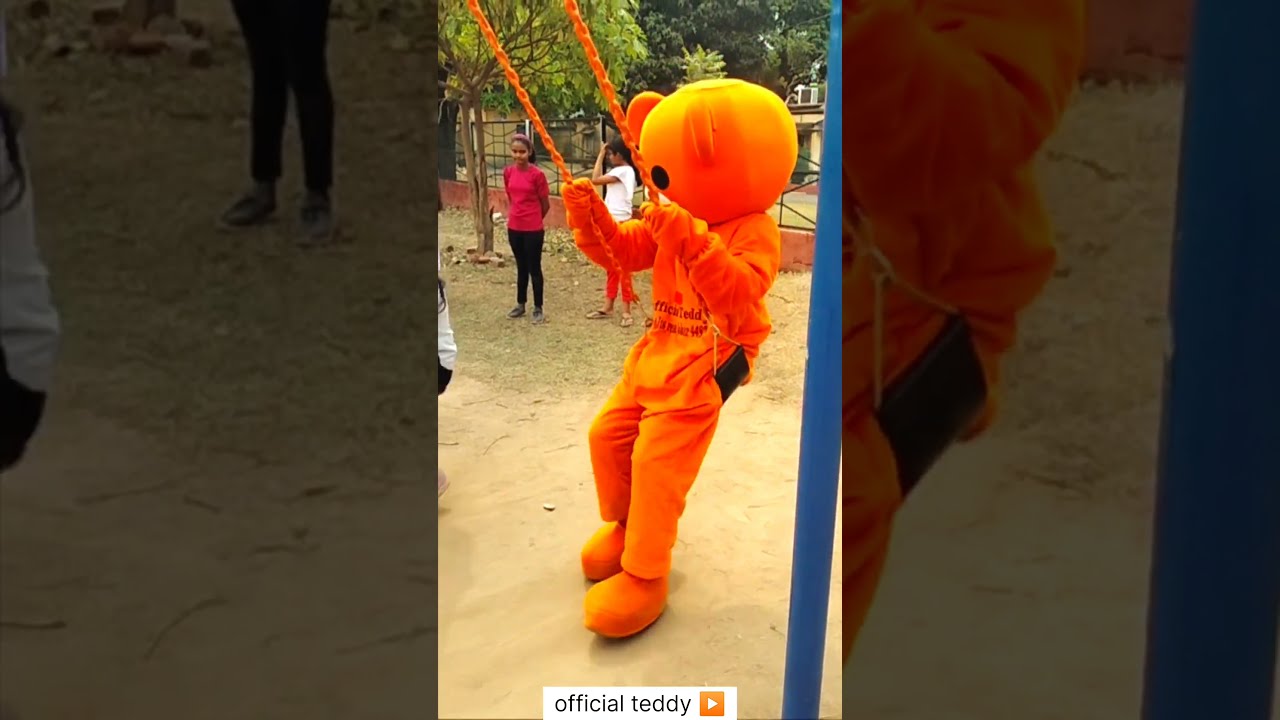In the center of the image, a bright, vertical photograph showcases a person dressed in an orange costume resembling a pumpkin, complete with orange ears and a black spot where the mouth would be. The figure is wearing an orange jumpsuit, matching boots, and is standing on sandy dirt. The character, identified as "Official Teddy," is holding onto an orange swing with chains extending upward and partially disappearing out of the frame. The swing's seat is black. Below the figure, a white square contains the words "Official Teddy" in black letters and features an orange square with an arrow pointing to the right.

Behind the costumed individual, two children are visible. One child has dark hair, brown skin, and wears a red shirt paired with black pants. The other child has black hair, a white shirt, and red pants. Behind them, a black metal fence topped with a row of bricks separates the scene from a background of trees, with one tree a darker green on the right and another, lighter green on the left.

The image is flanked by two tinted and blurred-out columns that zoom in on aspects of the main picture: the left column focuses on the feet of the child in the red shirt, while the right column zooms in on the swing. The overall composition resembles the shape of a high-definition TV screen divided into three sections, with the vibrant central image serving as the focal point.